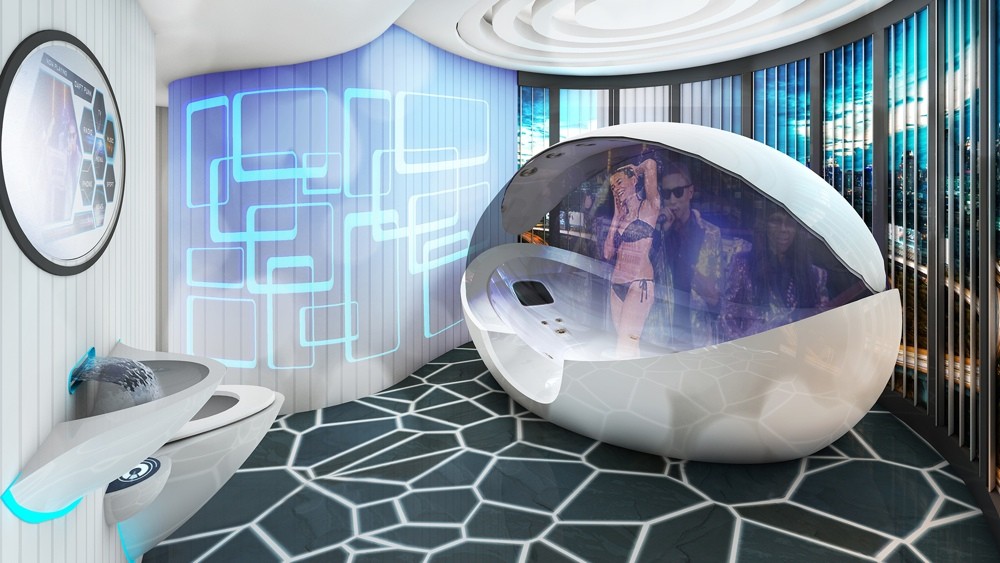The image showcases a highly futuristic room, with a prominent white, pod-like structure on the right half of the frame. This advanced pod, which resembles an egg or bathtub, has a reflective surface revealing a young woman in a black bikini inside, smiling with her arms raised. Alongside her are two men dressed in shiny suits; one wears sunglasses and holds a microphone. The pod appears to be part of a high-tech spa experience.

The left side of the image features a sleek white sink and toilet, which exude a futuristic design, accompanied by a mirror on the wall. The floor sports a dark greenish-gray hue, intricately patterned with intersecting white lines forming triangles and quadrilaterals. A circular image with hexagonal patterns seems to advertise various products.

Behind the pod, the curved wall adorned with vertical lines and light blue rectangles enhances the modern aesthetic. A large window on the right side of the wall reveals an urban cityscape bathed in neon lights and a descending sun, suggesting the time of day. The ambiance is both vibrant and serene, capturing the essence of a futuristic environment.